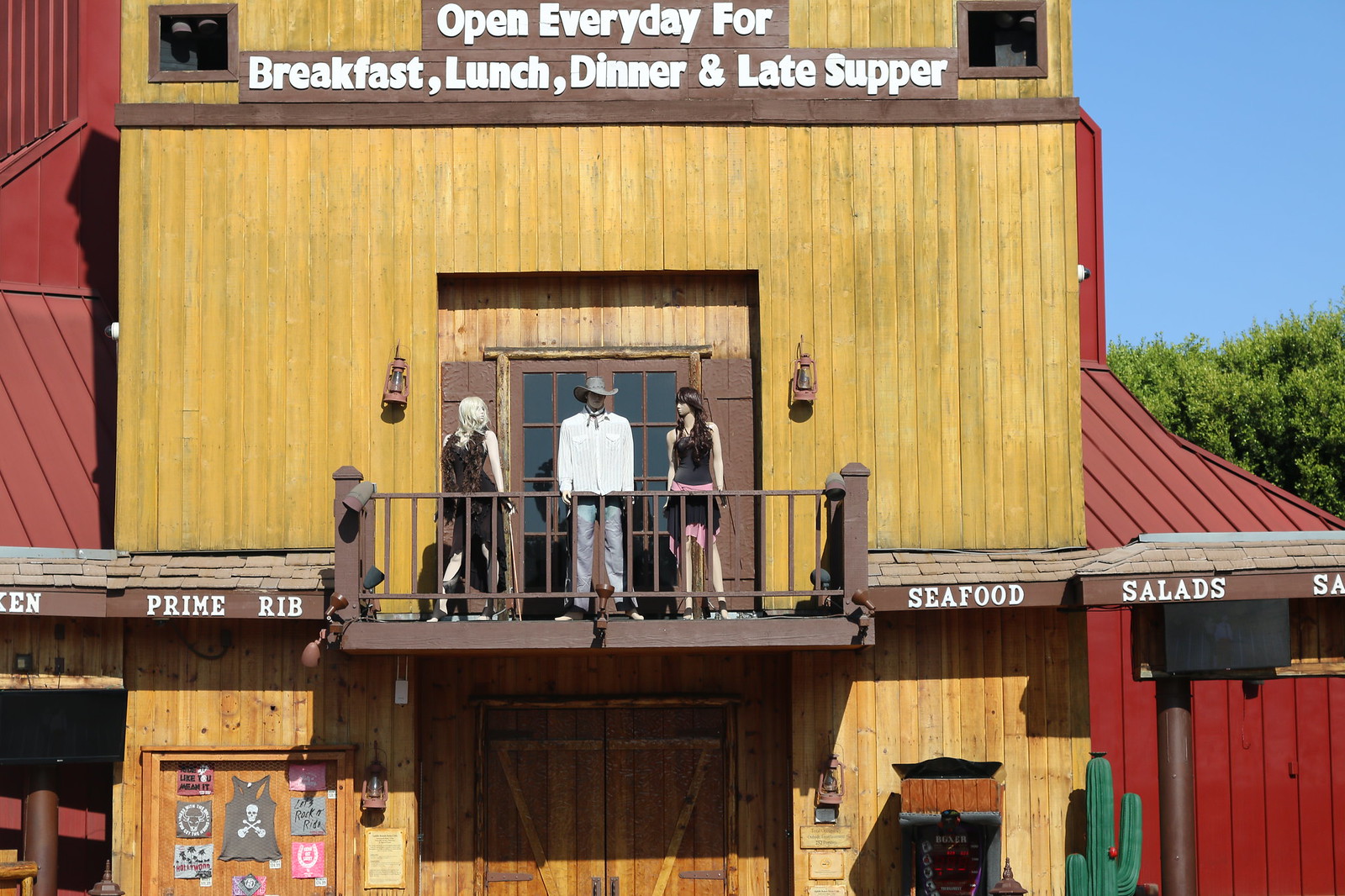This highly detailed, daytime color photograph captures a classic Old West-style restaurant or saloon with a distinct country-western vibe. The building's main face is adorned with vertical wooden slats painted beige, contrasted by red corrugated structures on either side. Atop the storefront is bold white text declaring, "Open Every Day for Breakfast, Lunch, Dinner, and Late Supper." Below this proclamation is an awning with additional text advertising prime rib, seafood, and salads.

A key feature of the building is its second-floor balcony, which sports a brown wrought iron railing. Strategically placed on this balcony are three mannequins dressed in period-appropriate Western attire. The male mannequin at the center is outfitted in a white long-sleeve shirt, jeans, and a cowboy hat, flanked by two female mannequins each wearing brown dresses, their poses suggesting they're looking off in different directions. 

The main entrance, situated at the bottom and center of the image, features sliding doors with brown trim above traditional barn-style doors. Adjacent to the entrance is a collection of merchandise, including T-shirts hanging on the door, and a small billboard posted to the bottom left of the facade displays various offerings. The scene is completed with a bright blue, cloudless sky and a distinctive cactus situated near the bottom right, contributing to the establishment's Southwestern ambience.